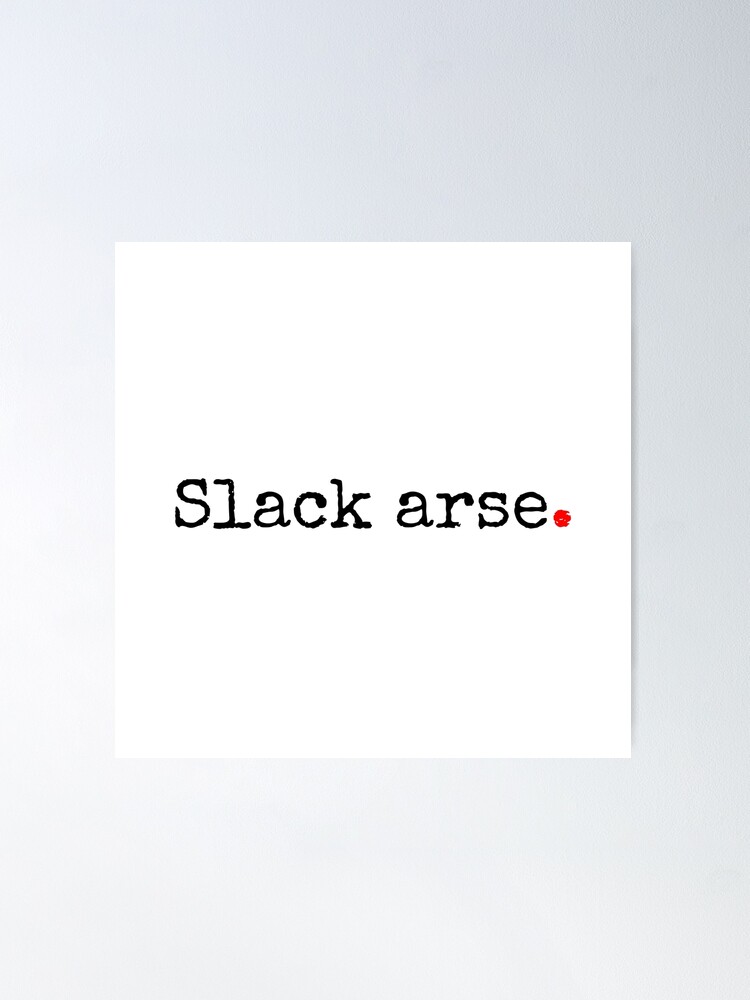The image features a white square resembling a post-it note, containing the text "SLACKARSE" in black typewriter-style font. A red period, appearing as if drawn with colored pencil, follows the word. This white square sits atop a large, solid gray rectangular background and casts a slight shadow on the right side, adding depth to the simplistic design.